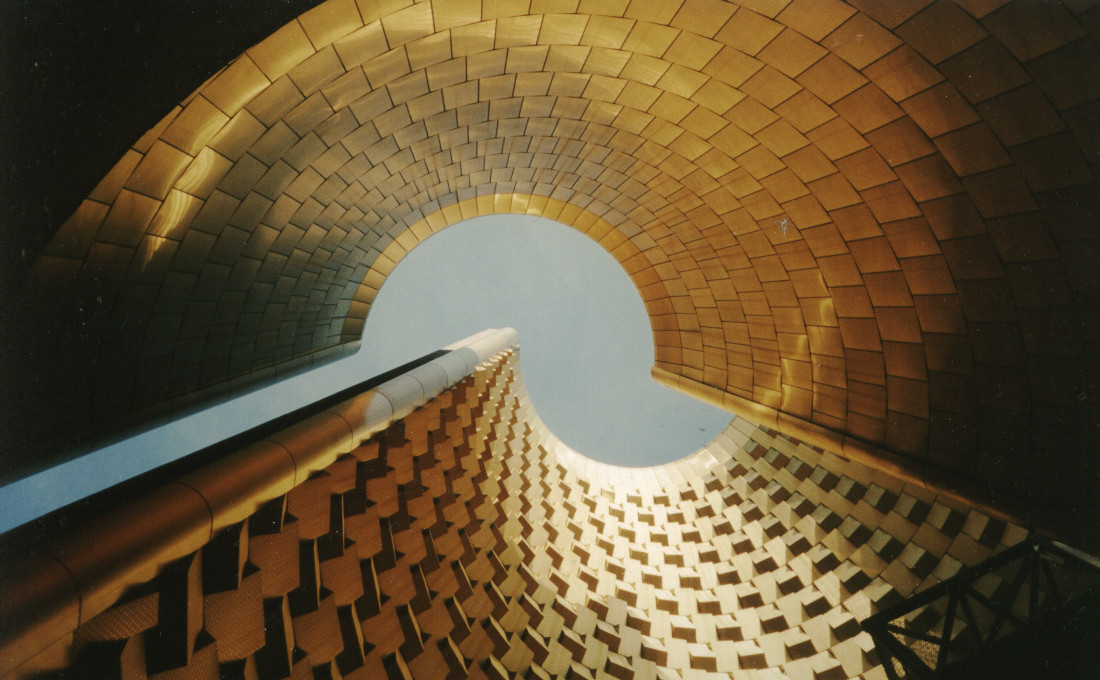The photograph captures a large, intricate structure consisting of two interlapped semicircular walls, creating a complex, tunnel-like formation that doesn't fully align. The wall in the top section of the image is constructed from multiple flat, tan-colored panels that transition into yellow panels at the top, forming a somewhat spiral dome shape. This top structure is positioned slightly to the left and descends inwards on its right side. The other wall, made from tan-colored stone blocks, features cylindrical, window-like projections and a woven texture of brown and white. On the right side of this segment, the structure curves back up behind the top wall, adding to the visual intricacy. At the bottom right corner, a black metal frame is visible, adding a finishing touch to this architectural marvel. The mismatched alignment and distinctive paneling and projections imbue the scene with a sense of dynamic, yet harmonious complexity.